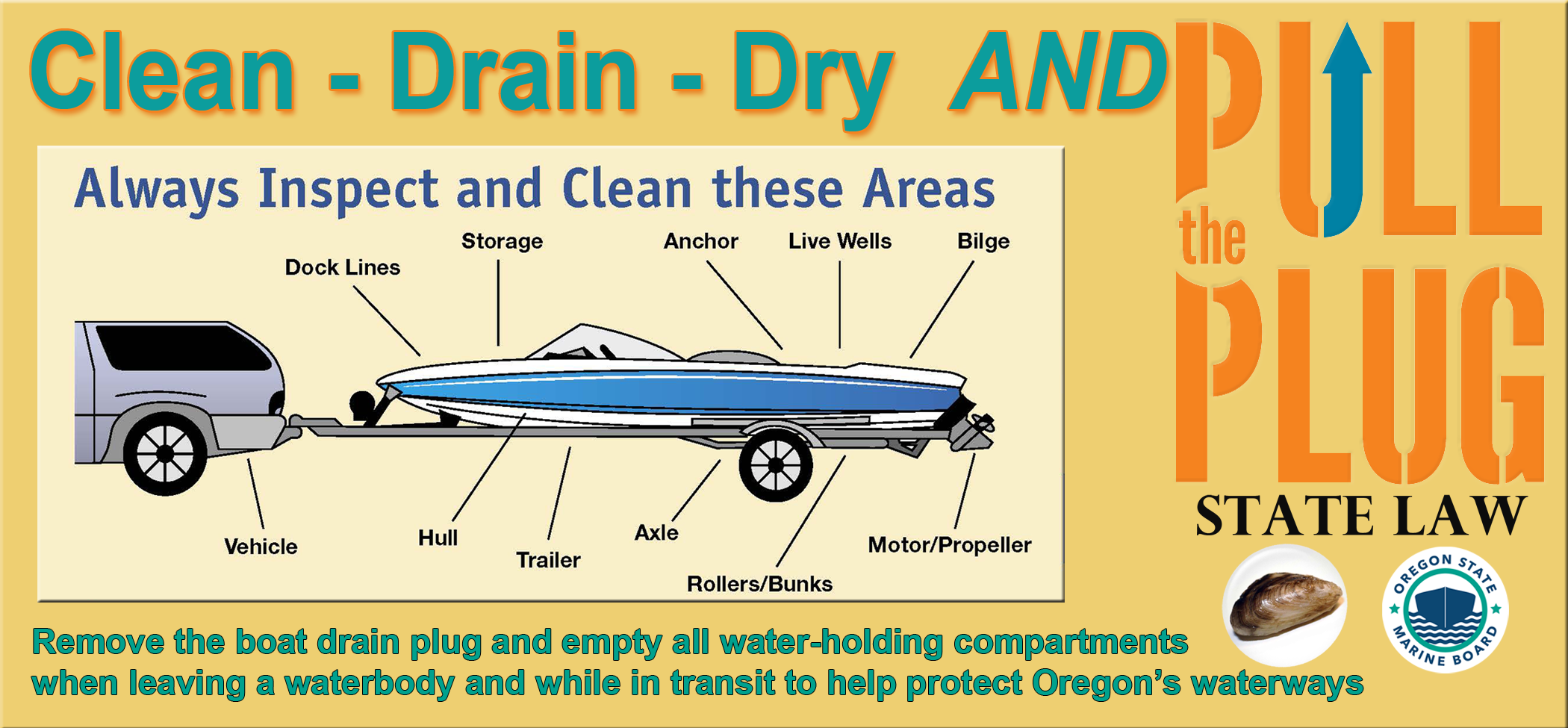This detailed poster, issued by the Oregon State Marine Board, serves as an educational advertisement about proper boat maintenance to protect Oregon's waterways. Set against a plain yellow background, the poster prominently features the text "Clean, Drain, Dry" in bold blue letters with a red outline, alongside "Pull the Plug" in a darker orange, with the right side of the 'U' forming an upward arrow in blue. Below this message, the poster declares "State Law" and incorporates the Oregon State Marine Board seal.

A central diagram illustrates a car towing a speedboat, highlighting various components with labels such as "dock lines," "storage," "anchor," "live wells," "bilge," "motor," "propeller," "rollers," "bunks," "axles," "trailer," "hull," and "vehicle." At the top of the diagram, it states "Always inspect and clean these areas." The bottom section of the poster advises boaters to "remove the boat drain plug and empty all water-holding compartments when leaving a water body and while in transit," emphasizing the importance of these actions to "help protect Oregon's waterways."